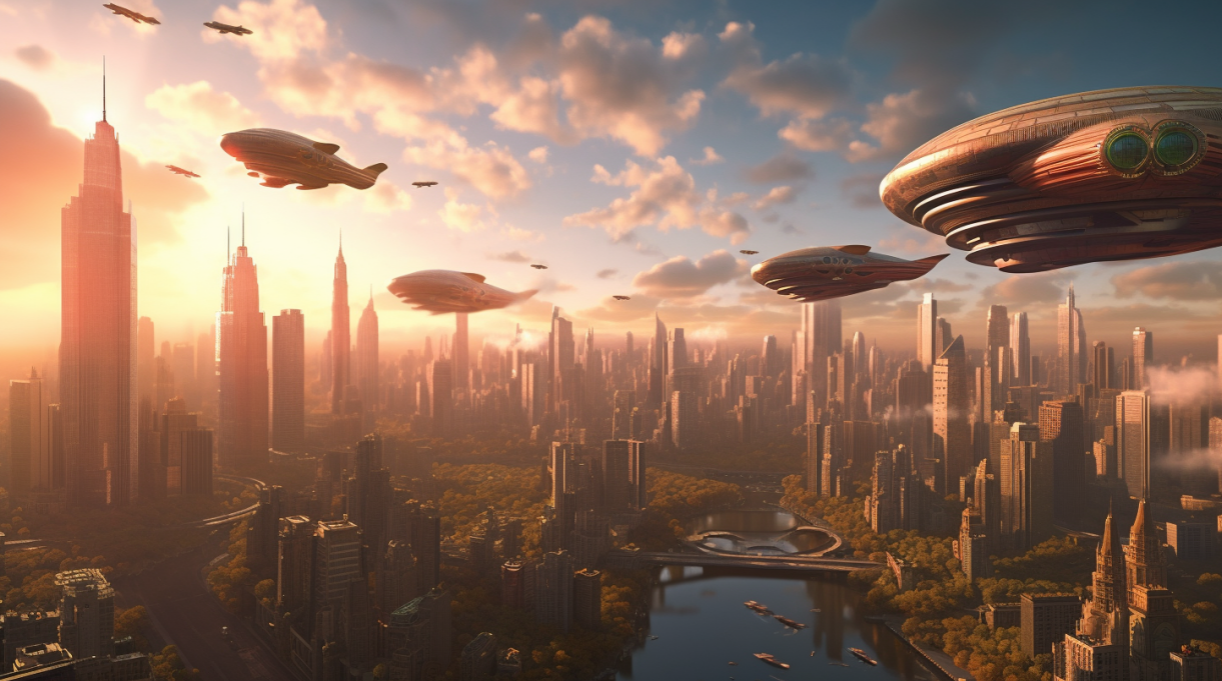The image portrays a highly detailed, futuristic cityscape that blends elements of New York and Chicago, possibly an AI-generated vision of the far future. Taken from an aerial perspective at sunset, the scene is bathed in warm light with a scattering of clouds. The sprawling metropolis is filled with towering skyscrapers that extend far into the horizon. These buildings, surrounded by abundant green spaces and interspersed with trees, reveal a significant emphasis on integrating nature within the urban landscape. Notably absent are traditional roads, replaced instead by a single, elevated monorail winding through the cityscape.

Prominent in the sky are numerous futuristic blimps or zeppelins—nine in total—along with sleek, oblong-shaped spaceships, possibly used for transport or something more ominous like an alien invasion. These airborne vehicles navigate the airspace, avoiding the skyscrapers effortlessly. In the center of the image, a river or inlet is spanned by a prominent bridge or highway, suggesting advanced infrastructure for both aerial and ground movement. The overall setting, with its blend of futuristic architecture and verdant expanses, evokes a sense of a meticulously planned, eco-conscious urban future.